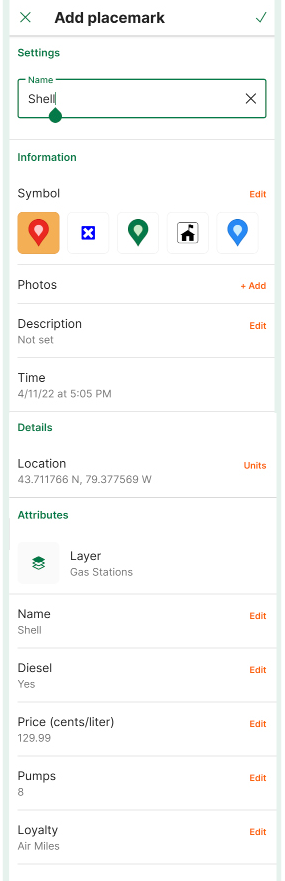The image is a screenshot of a GPS app interface. At the top of the screen, there is an option labeled "Add Placemark". Below this, there is a "Settings" button. The main section of the interface comprises various fields and options for adding detailed information about a location.

In the "Name" field, the user has typed "Shell". Following this, there are sections labeled "Information" and "Choose a Symbol" for further customization. Additional sections include options to add "Photos," a "Description," "Time," "Location," and "Attributes."

The "Attributes" section contains fields for more specific details such as "Name," "Diesel," "Price," "Pumps," and "Loyalty." All these fields appear to be organized under a broader "Details" section, with "Location" likely providing geographical coordinates or positioning information.

This detailed setup allows the user to comprehensively document and personalize a specific place on the GPS app.